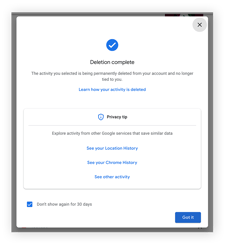A small fuzzy image is surrounded by a moderately thick black border. In the upper right-hand corner, a small gray circle containing an 'X' is prominently visible. The majority of the background is white space. At the center, a blue circle with a white checkmark stands out. Below this circle, centered in the frame, the phrase "Deletion complete" is written in black text.

Further down, in slightly smaller font aligned to the left, the text reads: "The activity you selected is being permanently deleted from your account and no longer...". The line breaks continue with "...tied to you." Centered and in blue text, another line reads: "Learn how your activity is deleted."

There is an expanse of white space beneath this text, followed by a small blue circle with an unclear label, likely saying "delivery tip" in black font. A faint horizontal line divides this section from the next.

In very light text, the message "Explore activity from other Google services that save similar data" is displayed. Below this, centered in blue text, are the options: "See your Location History" (with 'Location History' capitalized), "See your Chrome history" (with 'Chrome history' capitalized), and "See other activity."

To the left, a small blue square with a checkmark and the option "Don't show again for 30 days" in black text appears to have been selected. Finally, in the bottom right corner, a dark blue box contains the words "Got it" in white text.